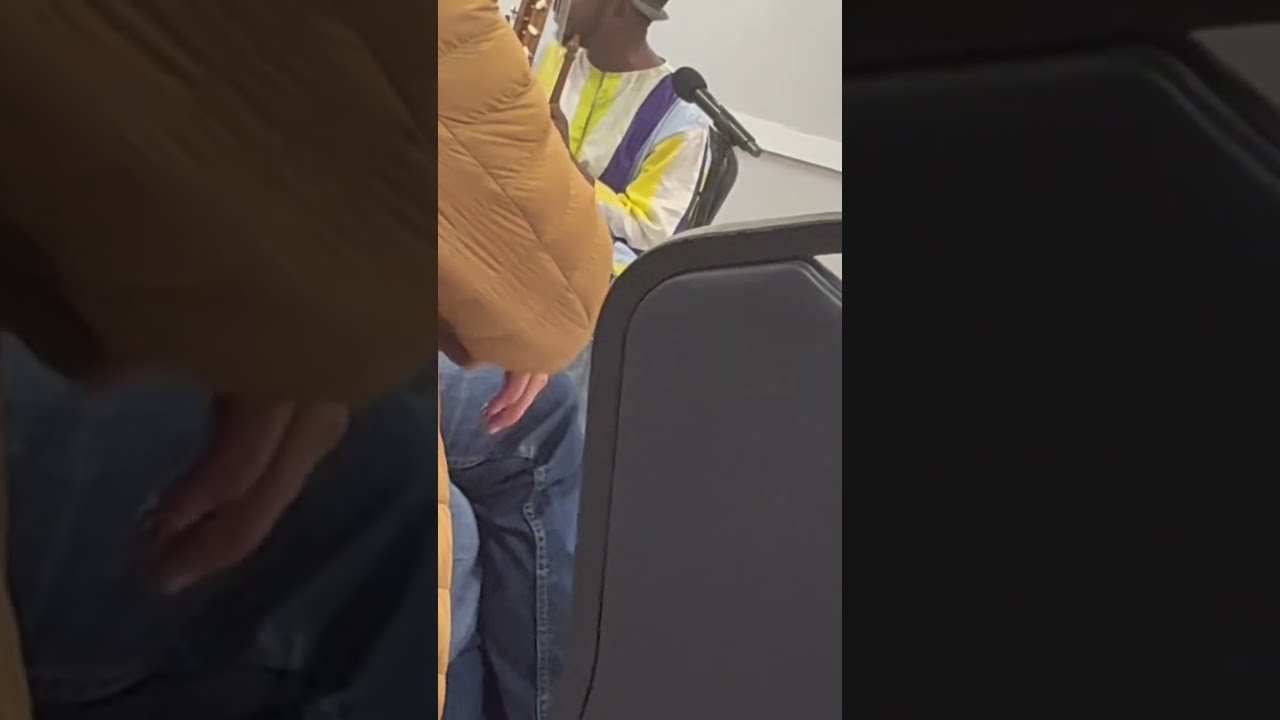In this detailed image, the central photograph occupies the middle vertical portion, surrounded by a backdrop, which is a darkened close-up of the center image. The main photograph depicts a scene inside a bus. A young black man, who seems to be wearing a white shirt adorned with yellow and possibly purple stripes, along with blue jeans, sits prominently in the foreground. He has a backpack on his back and a microphone stands nearby, suggesting he might be a singer. The man appears to be holding a guitar and also seems to be wearing a hat. To his left, another individual is visible, characterized by their thick orangey-brown or tan coat, with just their arm and hand exposed. This person's sleeve stands out, with fingers partially visible. The bus’s interior features a grey chair with a dark grey rim and a white wall in the background, enhancing the bus setting.